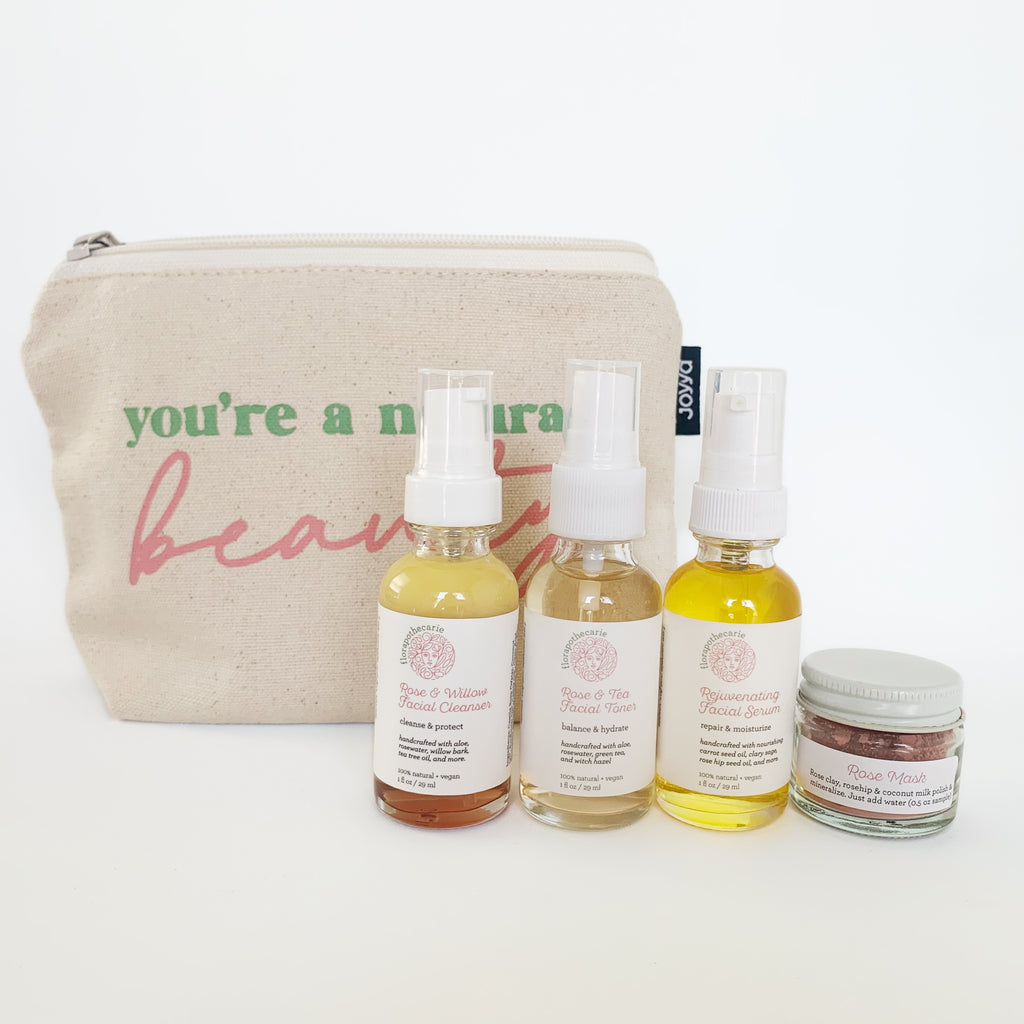This image displays a professionally photographed beauty kit set against a clean, white background, likely for an advertisement or promotional purposes. At the center of the composition is a natural, cotton drawstring bag featuring the phrase "You're a natural beauty" in green and pink fonts. Arranged in front of the bag are three elegantly designed dropper bottles and a small jar, each labeled with white stickers and pink lettering. The dropper bottles contain a facial cleanser, toner, and serum respectively, boasting descriptions like "cleanse and protect," "balance and hydrate," and "repair and moisturize." The smaller jar holds a rose mask made from a blend of rose clay, rose hip, and coconut milk, designed to promote a radiant complexion. The overall aesthetic emphasizes a commitment to natural, organic ingredients, appealing to consumers seeking wholesome beauty products.